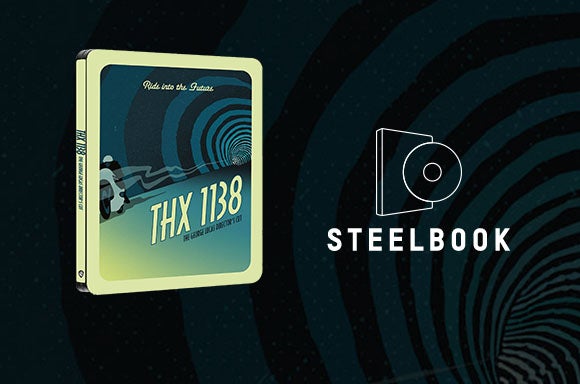This image serves as an advertisement for a Steelbook, featuring a multi-colored, striped background that visually resembles a tunnel or funnel with interspersed rings of black, dark green, and various shades of blue, progressively narrowing towards the bottom right corner. Positioned perfectly centered in the middle of the image are two key objects: on the left, there is a rectangular book or case labeled "THX 1138," displaying an image of the background itself, and on the right, an icon of a book cover paired with a circle enclosed by another circle. Below this icon, in all capital letters of a sans-serif font, is the word "Steelbook." The Steelbook case is meant for a movie, possibly a DVD or Blu-ray, and features a transparent white line drawing of a case with a disc. The artistic element also includes a cartoonish depiction of a person on a motorcycle with a white helmet, leaving a smoke trail, accentuated by the cylindrical tube design seen again within its imagery. The top of the image bears the text, "Ride into the future."